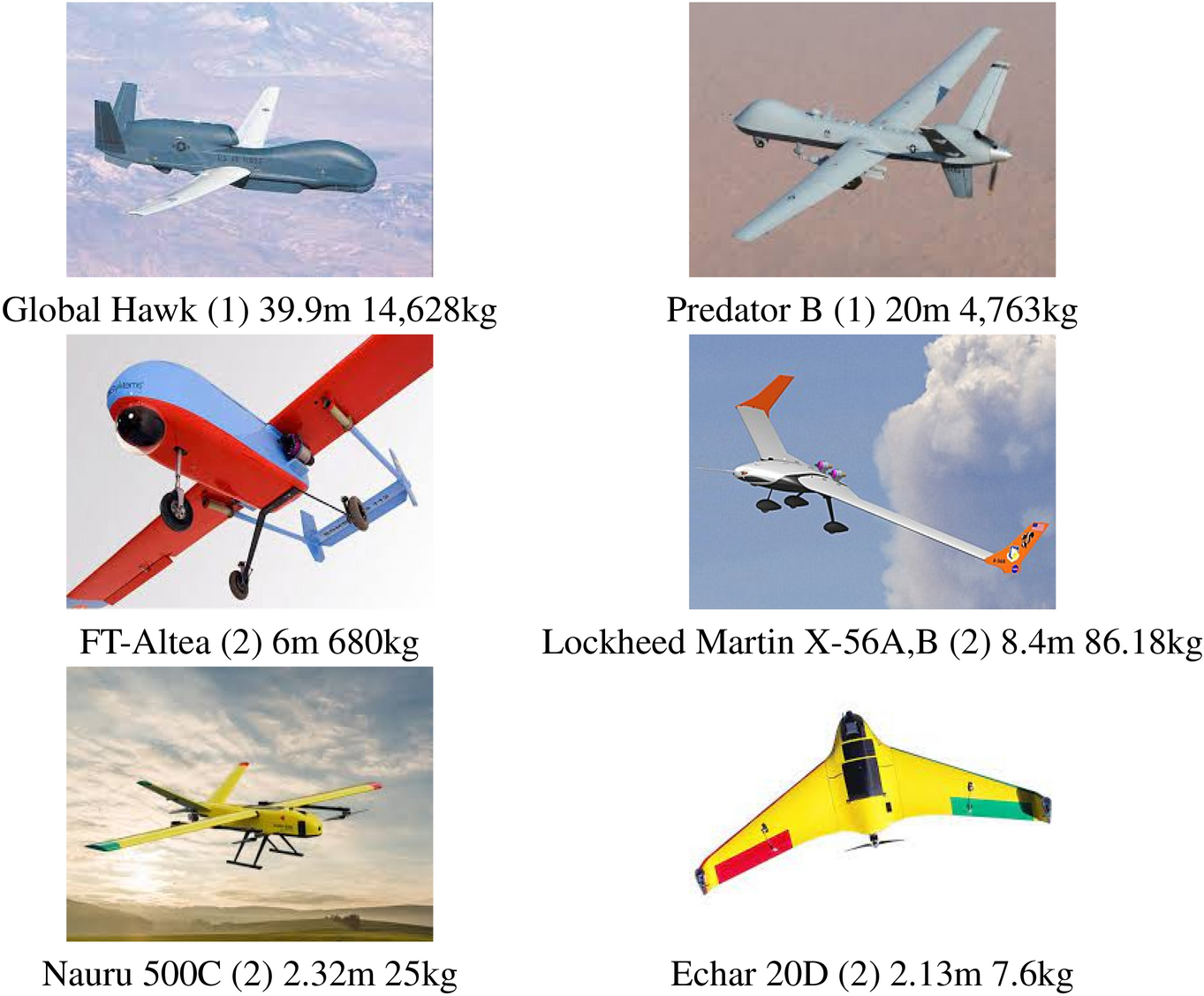The graphic presents a detailed display of six distinct aircraft types, arranged in two rows of three square images. Each aircraft is labeled with its name, dimensions, and weight in black text beneath the respective image. 

In the top row:
1. The first is a blue-and-white aircraft identified as "Global Hawk 1," measuring 39.9 meters and weighing 14,628 kilograms. This aircraft, with its significant size and military-like appearance, features a round front and white wings.
2. Next is a baby blue, red, and black aircraft known as "FT-ALTIA," which spans 6 meters and weighs 680 kilograms. It appears sleek with a combination of bright colors.
3. The third is a slender yellow aircraft accented with blue and red, labeled "Nauru 500C," with dimensions of 2.32 meters and a weight of 25 kilograms. 

In the bottom row:
4. The first aircraft here is a slightly pale grayish-blue "Predator B1," measuring 20 meters and weighing 4,763 kilograms. It is a larger, perhaps more industrial-looking plane.
5. The next is a silver and orange "Lockheed Martin X-56A, B," which measures 8.4 meters and weighs 86.18 kilograms. It features prominent orange tips on the wings.
6. Finally, there is a yellow and black aircraft with red and green accents, labeled "Ekar 20D," measuring 2.13 meters and weighing 7.6 kilograms.

The colors of the backgrounds vary, with some images featuring skies, adding to the vibrant and diverse color palette that includes various shades of blue, grays, and neutrals. The detailed captions under each image provide a clear and informative insight into the specifications and appearances of the aircraft, making this graphic a comprehensive guide to these six distinct planes.